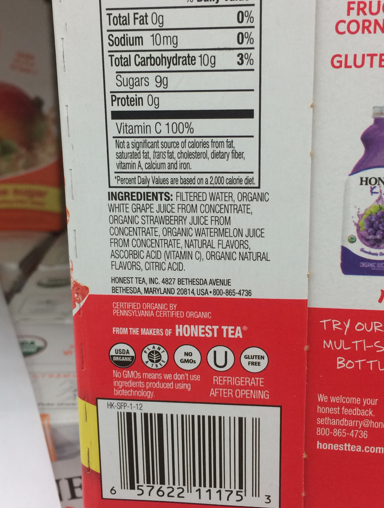This detailed close-up photograph captures the back of a square container prominently displaying its nutritional label and ingredients. The container exhibits a white top transitioning into a red bottom, adorned with black, white, and red writing. At the center top of the label, a nutritional table in black writing lists the calories and nutrients, while the ingredients are detailed below in black text. These include filtered water, organic white grape juice from concentrate, organic strawberry juice from concentrate, organic watermelon juice from concentrate, natural flavors, ascorbic acid (vitamin C), organic natural flavors, and citric acid. Just under the ingredients, the label features logos and text with a red background, indicating the product is from the makers of Honest Tea. 

In the top right corner of this image, red text stands out, likely a call to attention. Further down, a plastic bottle with a purple logo is visible, alongside a sticker featuring blue grapes and a message inviting honest feedback on the website honesttea.com. A barcode, presented in a white rectangle outlined in black, is located at the bottom center of the image. Below the barcode, there is some additional white writing. The left edge of the image includes some out-of-focus white, red, and yellow containers in the background, providing contextual depth.